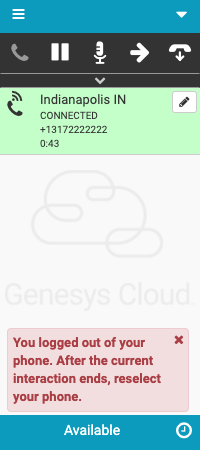The top of the image features a dark blue border. Directly beneath it, a black border contains several icons: a phone headset icon, a pause icon, a microphone icon, a right-pointing arrow, and another phone headset icon with a downward-pointing arrow beneath it. Below this black border, a horizontal line separates it from the subsequent elements.

Further down, a green box is positioned with a phone headset icon emitting sound waves on its left side. To the right of this green box is a white box centered with a pencil icon. The text within the green box reads, "Indianapolis IN Connected, plus 1317222043."

Below the green box is a gray box labeled "Genesis Cloud." Directly underneath, a pink box contains the message: "You log out of your phone after the current interaction ends, reselect your phone."

Finally, at the bottom of the image, a blue box displays the word "Available" in its center.